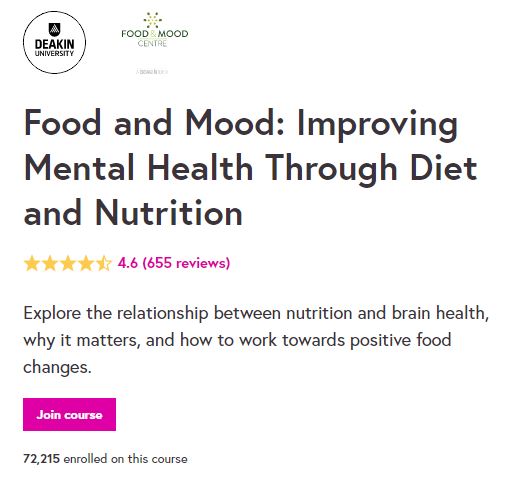The image is predominantly white, with various sections of black text and a notable absence of any border, giving it a clean, minimalist appearance. The content is structured within what appears to be a square frame. 

In the upper left corner, there's a black circle featuring a white center, containing the text "Deakin University." To the right of this emblem, the words "Food & Mood Centre" are displayed in green. Dominating the upper section is a bold, black headline stating, "Food and Mood: Improving Mental Health Through Diet and Nutrition," accompanied by a rating of 4.6 stars, followed by "(655 reviews)" in parentheses.

Below the headline, more black text invites the reader to "Explore the relationship between nutrition and brain health, why it matters, and how to work toward positive food changes." Beneath this explanatory text, a bright fuchsia rectangle with the words "Join Course" serves as a call-to-action button for those interested in enrolling and learning about nutrition's impact on mental health.

At the very bottom, in small black text, the image notes that "22,215 enrolled on this course," highlighting its popularity and the credibility of its academic affiliation.